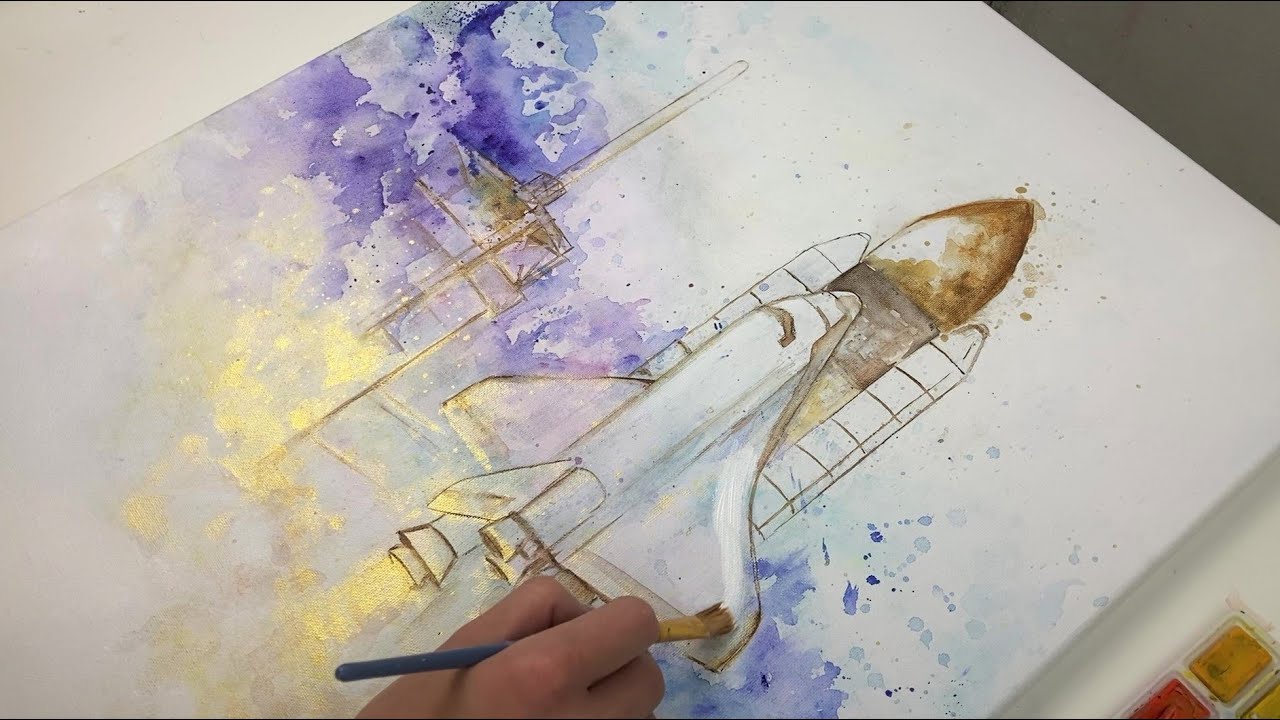The image captures a detailed scene of someone engaged in painting on a flat white canvas, likely placed on a table or counter. The artist uses a blue-handled paintbrush with a gold ferrule and brown bristles to intricately paint the body of a space shuttle white. This space shuttle, which features a streamlined design with wings swept back akin to an airplane, is depicted in a dynamic ascent. Propelled by three rocket boosters, the craft emits a striking gold thrust instead of traditional flames. The sky in the painting shifts from a deep purple at the bottom to white at the top, providing a dramatic backdrop. In the bottom right corner of the image, small yellow and red paint cartridges are visible, adding a touch of color and context to the creative process. A human hand, positioned slightly to the left of the canvas, is seen in action, diligently adding details to the space shuttle's body.